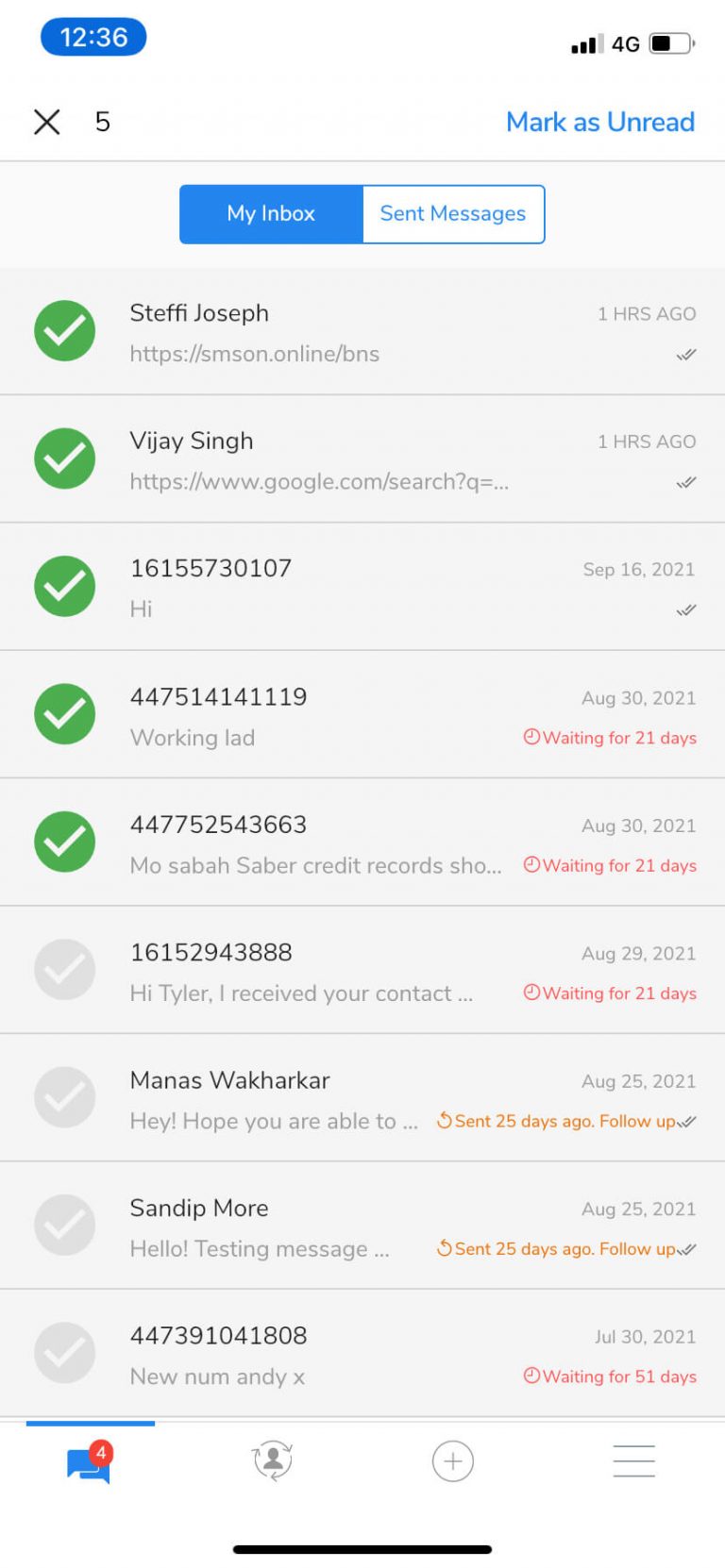A detailed screenshot of a smartphone's email inbox is displayed. At the top, the status bar shows the time "12:36," a 4G logo, and a battery icon indicating 50% charge. Below the status bar, there is a blue bubble with the number “5” to the right and a cross-out "X" icon, followed by an option marked "unread."

The inbox interface is divided into sections. The top section features two selectable tabs: "Inbox" highlighted in blue and "Sent Messages" adjacent to it. Below these tabs, email entries are listed in a gray-shaded area, each accompanied by a check mark to the left.

1. **Steffi Johnson** - One hour ago: This email has a green circle with a white check mark.
2. **Vijay Singh** - One hour ago: Similar to the first email, it also has a green circle with a white check mark.
3. **16155730107**: The email listed with this number shows a green circle with a white check mark.
4. **447514141119** - August 30, 2021: Displayed with a red message stating "waiting for 21 days" and a green circle with a white check mark.
5. **447752543663** - August 30, 2021: Also shows "waiting for 21 days" in red and a green circle with a white check mark.
6. **16152943888** - August 29, 2021: Marked "waiting for 21 days" in red, but without a check mark.
7. **Manas Wakarkar** - August 25, 2021: Displayed with a refresh arrow icon and the message "sent 25 days ago, follow up" in red, with no check mark.
8. **Sandip Moore** - No check mark, with a refresh arrow and the message "sent 21 days ago, follow up."
9. **447391041808** - July 30, 2021: This entry shows "waiting for 51 days" in red text with no check mark.

At the bottom of the inbox display are further icons: a conversation bubble indicating four messages, a user ID icon, a plus sign inside a circle, and a hamburger menu icon on the right.

This detailed visual inspection provides a comprehensive view of the email interface, revealing both read and unread messages along with their statuses and timestamps.